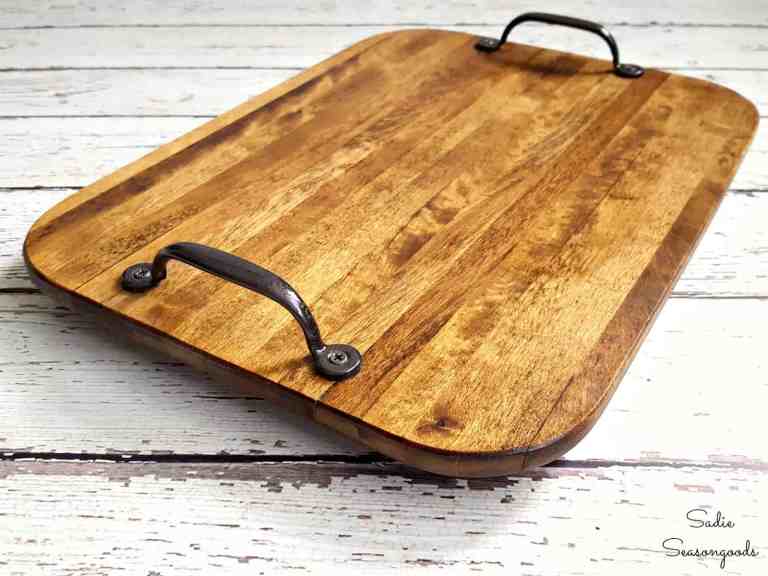This photograph, created by Sadie Seasongoods, features a richly detailed scene of rustic charm. Central to the image is a thick, rounded rectangle-shaped wooden tray, evocative of a charcuterie or cutting board, boasting a warm, rich brown hue. Crafted from multiple strips of wood seamlessly pieced together, the tray’s depth exceeds an inch, with gracefully rounded edges and corners. Enhancing its functionality, two almost black metal handles, securely fastened with Phillips head screws, flank each side. The tray rests on a weathered, white-painted wooden table that recalls a picnic table, showing the natural brown wood beneath through distressed spots. The table's slats run horizontally and contribute to the overall rustic aesthetics. At the tray’s bottom right corner, in elegant black script, is the artist's name, "Sadie Seasongoods," subtly enhancing the personal touch of this beautifully captured still life.